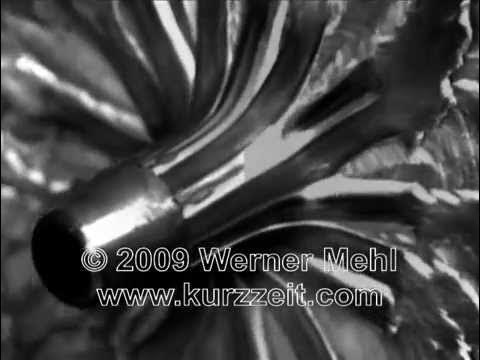This black and white image features a mechanical device with a detailed, metallic structure. Central to the image is a metal component that resembles the end of a light bulb or perhaps an intricate piece of equipment featuring fluted, fan-like sections that splay outwards, much like the shape of an octopus or an open umbrella. The device appears to have a zigzag indentation design that encircles it, with parts highlighted in bright white and shaded in deep black, adding a three-dimensional texture to the piece. Against the predominantly grayish and silver tones, the image bears the watermark "Copyright 2009 Werner Mell, www.curzett.com" at the bottom, although the overall picture is slightly blurred, making finer details hard to discern. The background maintains a blurred, rectangle-shaped space, emphasizing the focus on the central metal apparatus.